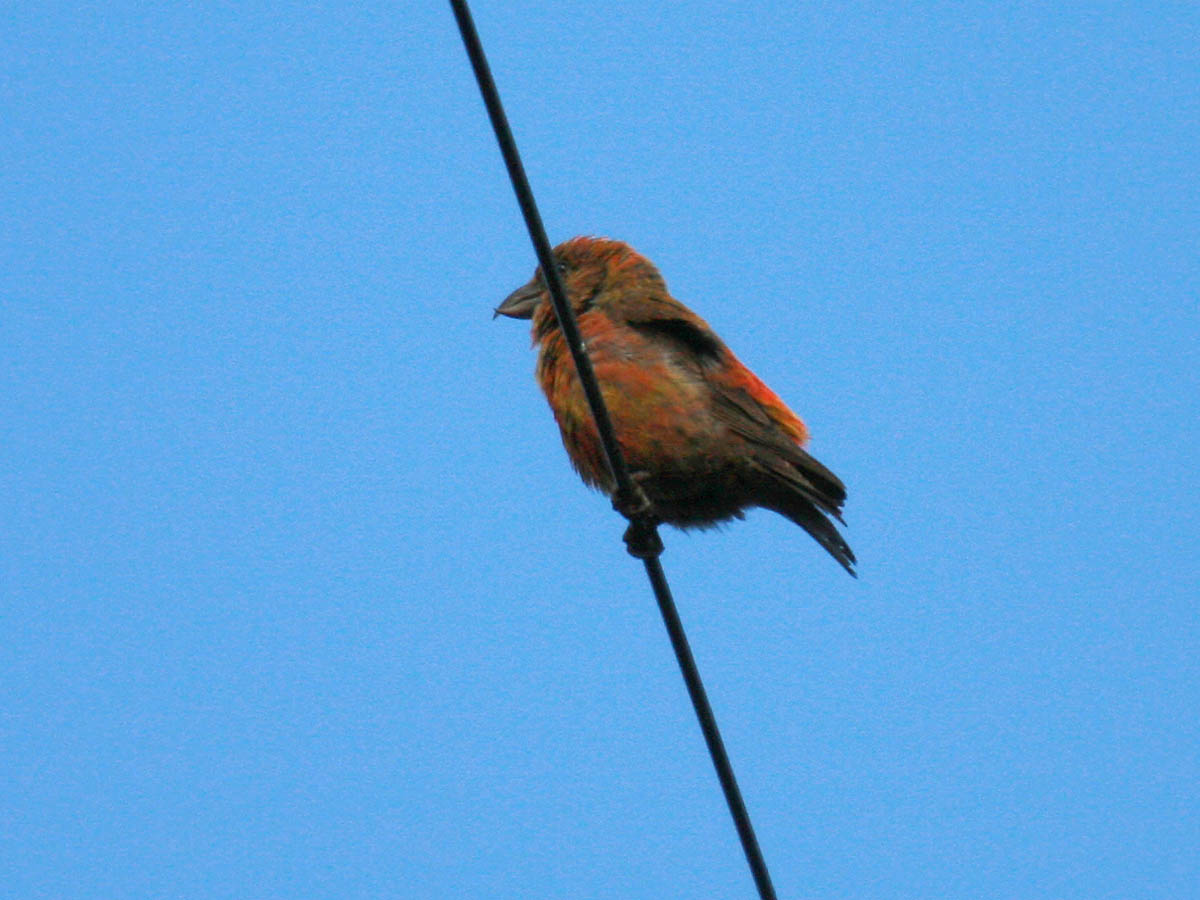The image showcases a single small bird perched on a wire against a perfectly clear blue sky with no clouds. The wire cuts across the center of the photo from top to bottom, framing the bird right in the middle, horizontally and vertically. The bird, facing left, features a striking combination of orange, red, and black hues. Its body feathers transition from reddish to orange with some patches of brown and gray. The bird's tail feathers are dark, and its black beak and feet are clearly visible. The angle of the photograph is slightly from below, making the bird's eye partially obscured by the wire. The backdrop is an uninterrupted expanse of blue, ensuring the bird remains the focal point of this minimalist composition.